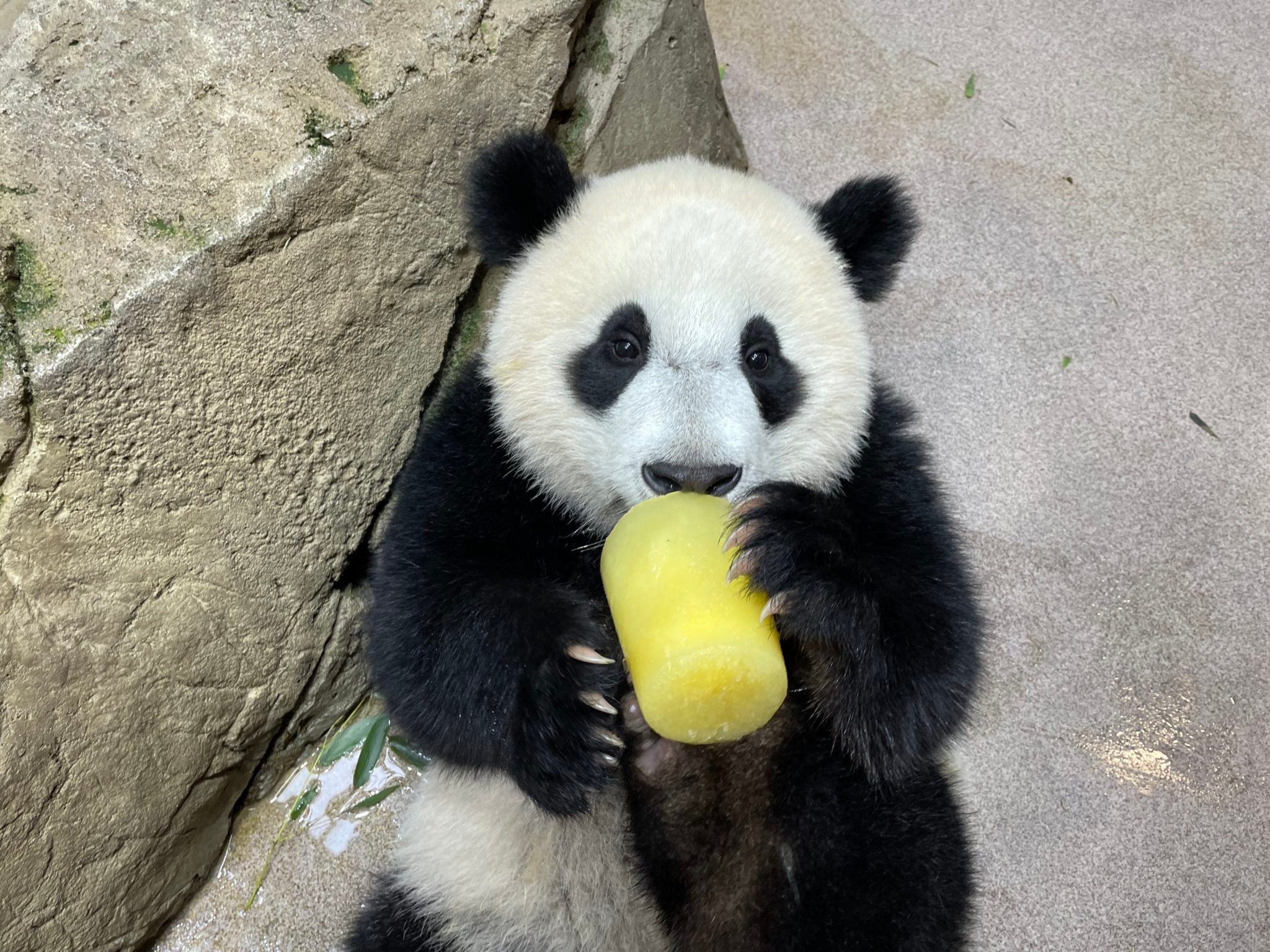This photograph captures a baby panda with a small frame, occupying the center of the image. The panda is standing slightly lower in the frame, with its legs partially cut off at the bottom. Its appearance is characterized by a white, round head adorned with black ears, black eye markings, and a black nose. The panda's body features black upper limbs and a white midsection on one side.

The panda is grasping a yellow cylindrical object, which appears to be similar to a shaved piece of bamboo or a frozen natural juice bar, with both its clawed hands and a foot placed underneath. The object is raised to the panda's mouth, as if it's biting or licking it. Its black paws are clearly visible, extending sharp claws around the item.

The backdrop consists of a natural stone wall, predominantly gray with patches of green moss, and a large boulder behind the panda that has a notable diagonal crack. The scene adds a rustic, nature-oriented feel to the photograph. The baby panda's innocent and somewhat shy expression is directed straight at the camera, making the image both charming and endearing.